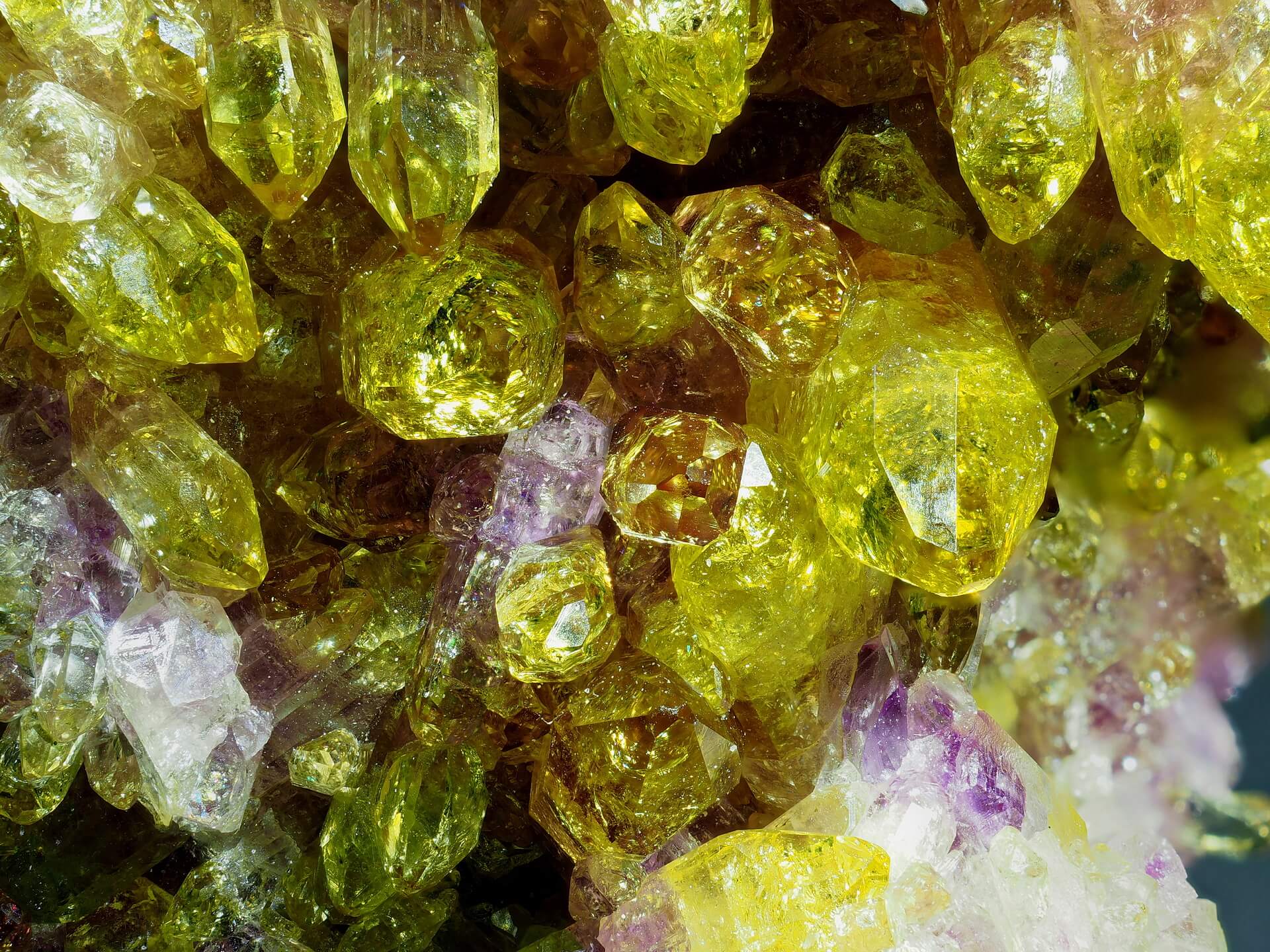This close-up photograph captures a stunning array of crystal formations. Dominating the scene, the crystals are primarily a vibrant yellow with hints of green, interspersed with patches of purple and white. The cluster resembles the inner core of a geode, where numerous crystal arms jut out in various directions—some extending towards the viewer and others angled perpendicularly. The overall effect is a dense, shiny amalgamation that completely fills the frame, set against a stark black background which emphasizes the vivid colors. Centrally, a significant piece features a mix of yellow, purple, and white, with a large green crystal boasting a round space near the top right. Beneath this centerpiece, a concentration of crystals in lighter hues, almost snow-like, can be seen. Several other smaller formations, including a light purple amethyst-like one, add depth and variety to the ensemble. No text, watermark, or context is provided, allowing the intricate beauty of the crystals to take center stage.